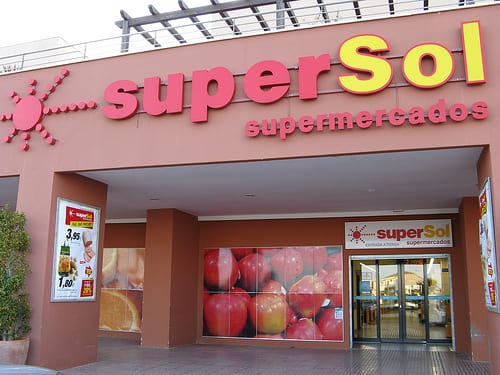This color photo, taken outdoors during the daytime under an overcast sky, captures the front entrance of a supermarket named "Super Sol Supermercados," with the sign displayed prominently in large letters. The word "Super" is in red, "Sol" is in yellow, and "Supermercados" is in red below. The design around the windows and signage includes a blend of lavender, tan, and brown colors. 

The entryway features double glass sliding doors that are motion-activated. Flanking these doors are large posters showcasing various produce. On the left side, there is a grand image of red apples, followed by a mural of citrus fruits. Adjacent to these posters, on a supporting wall, are advertisements that seem to highlight sales items.

Further to the left, another supporting beam also hosts sales information, reinforcing the emphasis on promotional deals. The architectural elements include beige support structures, adding to the store's aesthetic. The overall scene depicts a vibrant and inviting supermarket entrance, adorned with colorful signage and fresh produce imagery, effectively inviting customers into the "Super Sol Supermercados."